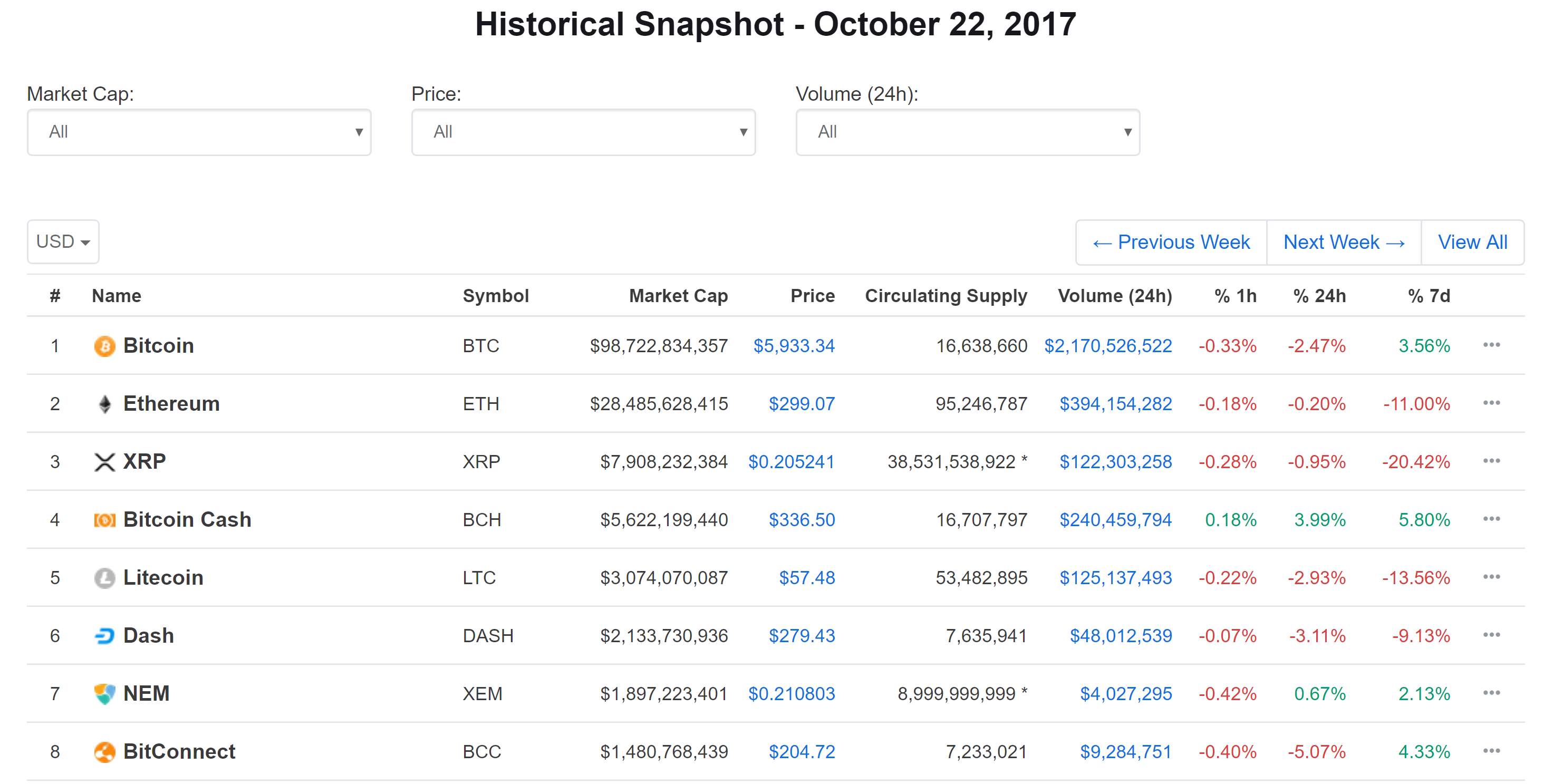The image portrays historical price data for various cryptocurrencies, set against a plain white backdrop. Titled "Historical Snapshot, October 22nd, 2017" in black font at the top, this image dates back to an early period in cryptocurrency history. The snapshot presents detailed information for eight cryptocurrencies: Bitcoin (BTC), Ethereum (ETH), XRP (XRP), Bitcoin Cash (BCH), Litecoin (LTC), Dash (DASH), NEM (XEM), and BitConnect (BCC).

At the forefront, Bitcoin (BTC) is highlighted with a market capitalization of approximately $98 billion and a price of $5,933.34 per coin. The table also includes columns for circulating supply, 24-hour trading volume, and percentage changes over one hour, 24 hours, and seven days. Notably, many of the percentages show declines, indicating a period of downward trends across the market.

Despite the lack of information about the specific application used to acquire this data, the image offers a comprehensive view of the cryptocurrency landscape, reflecting broader market sentiments at that time.